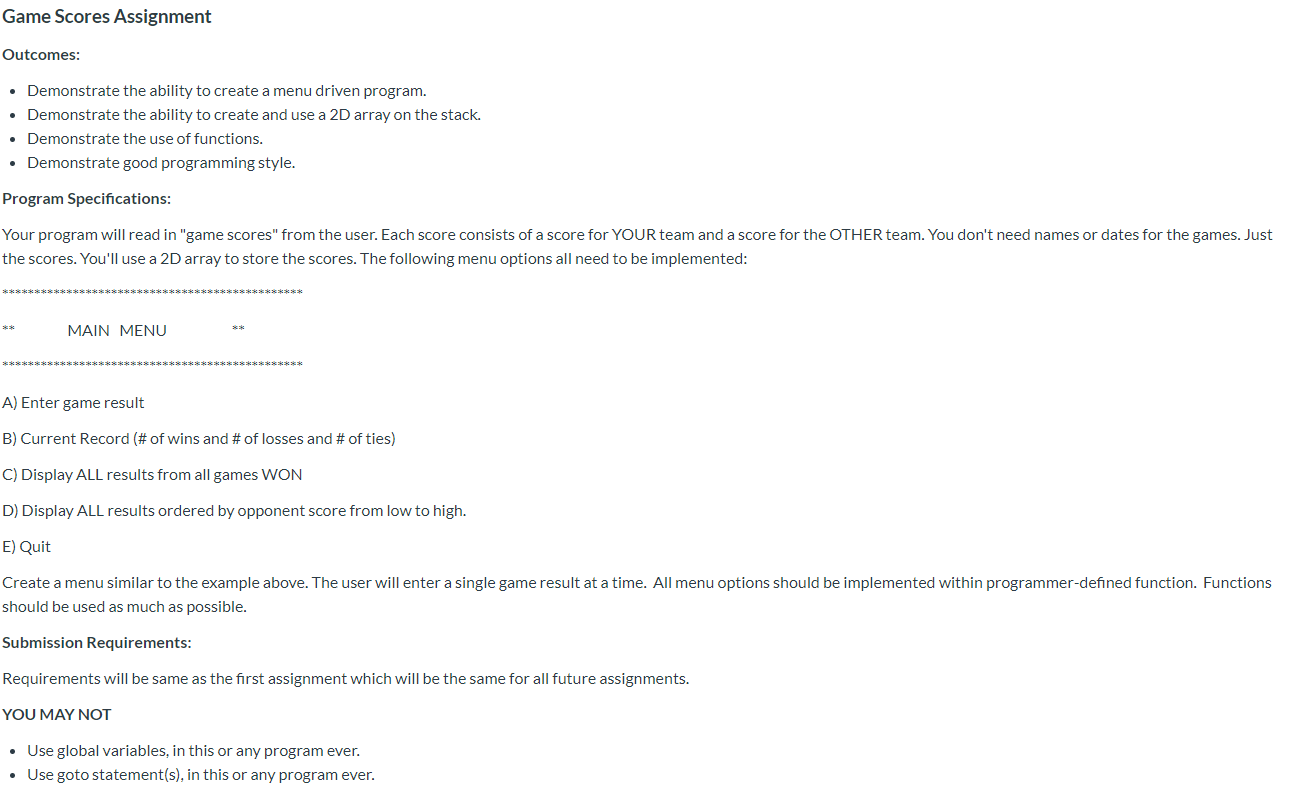The image is a screenshot of a webpage detailing an assignment for a programming class. At the top of the webpage, the title "Game Scores Assignments" is prominently displayed in black text. Beneath this title is a section labeled "Outcomes," listing objectives for the assignment: "Demonstrate the Ability to Create a Menu-Driven Program," "Demonstrate the Ability to Create and Use a 3D Array on the Stack," "Demonstrate the Use of Functions," and "Demonstrate Good Programming Style."

The next section, titled "Program Specifications" in bold black font, gives a detailed description of the task. The program requires reading game scores from users, with each user inputting scores for both their team and the opposing team. Names and dates for the games are not needed; only the scores are necessary. These scores should be stored in a 2D array.

The assignment outlines a menu system with various options, highlighted by asterisks surrounding "Main Menu." The menu options listed are:
- A: Enter Game Results
- B: Current Record
- C: Display All Results for All Games